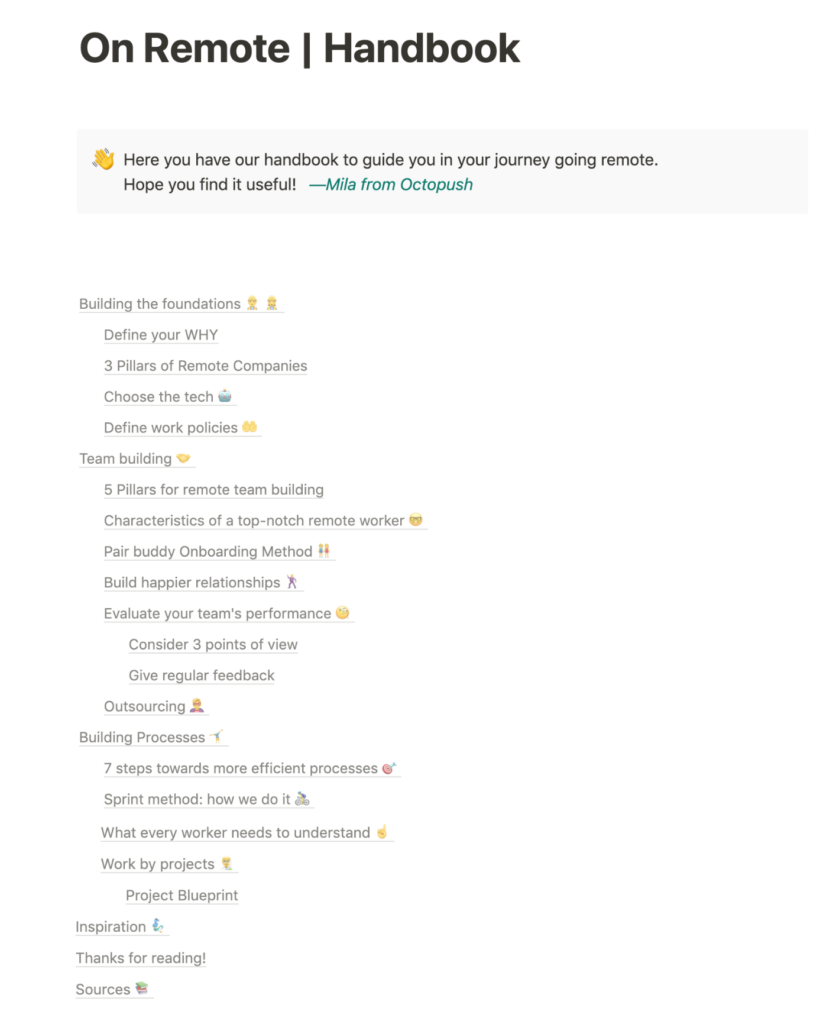This image is a screenshot from an unidentified digital device, such as a desktop, tablet, laptop, or smartphone. The uncertainty comes from the image being cropped on the left, right, top, and bottom edges.

At the top of the screenshot, a bold black banner reads "On Remote," followed by the word "Handbook" also in bold black text. Below this, a gray pop-up box, seemingly from Google, features an orange and yellow hand icon with blue bands around it. Within this box, regular black text states: "Here you have our handbook to guide you in your journey going remote. Hope you find it useful." The message is signed off with "Myla, from Octopush," which is italicized, clickable, and might be teal in color.

Beneath the pop-up, the content expands into a cascading menu format teeming with comments and various emojis. Key topics and points include:

- "Building a Foundation," featuring a male and female emoji.
- "Define Your WHY" with WHY in all caps.
- "Three Pillars of Remote Companies."
- "Choose the Tech" illustrated by a robot emoji.
- "Define Work Policies" shown with two hands icon.
- "Team Building" with a handshake emoji.
- "Characteristics of a Top-Notch Remote Worker," accompanied by a geeky face emoji.
- "Pair Buddy Onboarding Method," shown with emojis of two people, one in a blue shirt and the other in a red shirt.
- "Build Happier Relationships," represented by a person wearing a purple pantsuit.
- "Elevate Your Team's Performance," with an emoji wearing a monocle over the right eye.
- Additional sections on "Consider Three Points of View," "Give Regular Feedback," and "Outsourcing," showing a person in a purple shirt with blonde hair.
- "Building Processes," depicted with a person stretching out their arms, wearing a blue shirt and dark blue shorts.
- "Seven Steps Toward More Efficient Processing," featuring a target with a red center and blue arrow.
- "Sprint Method: How We Do It," represented by a person on a gray bike, sporting a light blue shirt, shorts, and helmet.
- "What Every Worker Needs to Understand," with a one-up finger-pointing icon.
- "Work by Projects," shown with a person in a cyan blue shirt.
- "Project Blueprint Inspection," featuring a person looking down, seated on a desk edge, wearing a dark blue shirt and teal shorts.

The screenshot concludes with "Thanks For Reading!" followed by "Sources" illustrated with stacked books colored green, red, and blue.